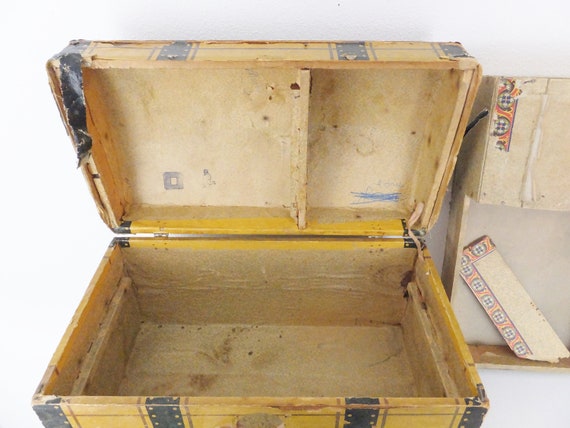The image depicts an open, old wooden chest with its lid tilted back on hinges. The interior of the chest is empty and lined with a cream-colored overlay that appears to be contact paper designed to mimic wood. The exterior of the chest is a yellowish wooden color adorned with black perforated film strip-like patterns, adding an aged and worn aesthetic. The corners of the box are reinforced with small silver brackets, hinting at its durability. To the right side of the photograph, part of another wooden structure is visible, resembling a frame that stands vertically, though its exact nature is unclear due to some visible damage or broken sections. The overall impression is that of a vintage, potentially handmade item, possibly a cigar box, designed to evoke nostalgia and history.